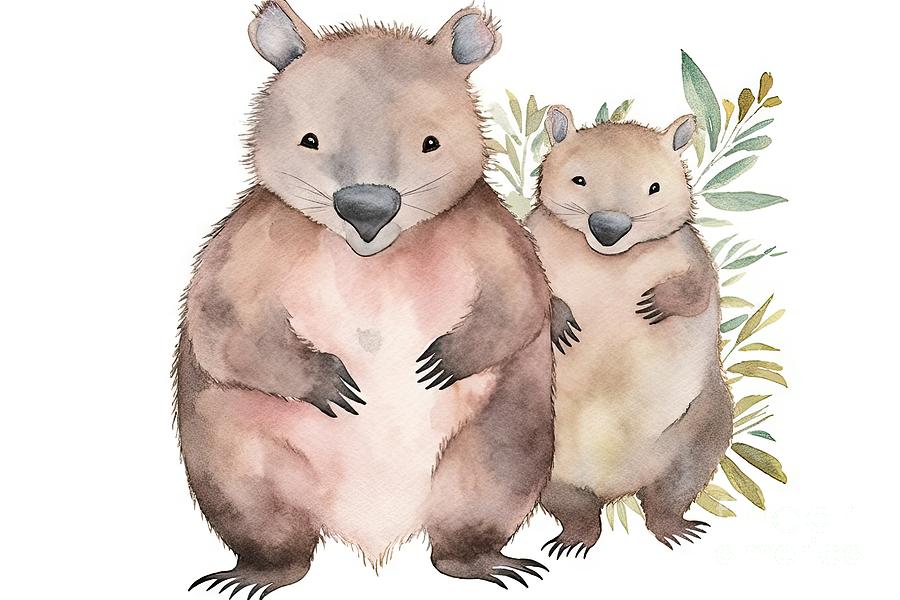This captivating hand-painted illustration, possibly rendered in gouache or watercolor, could be an enchanting page from a children's book. It features two charming animals that resemble mole-like or hedgehog-like creatures, standing side by side in a serene and detailed scene. The larger creature on the left exhibits a reddish-brown hue with gray ears, a gray nose, and dark button eyes, alongside sharp claws and feet adorned with six toes on one foot and five on the other. The smaller companion, with a lighter brown coat and a similar friendly expression, appears to be a younger version, possibly suggesting a parent-child relationship. Both creatures have distinct whiskers extending from their black noses and possess five fingers. The artwork is enriched with a palette of beautiful shades of brown, red, and green, highlighting the detailed tinting and tonal variations that bring the scene to life. Background greenery in muted watercolor tones adds to the tranquil and endearing atmosphere of this beautifully illustrated moment.